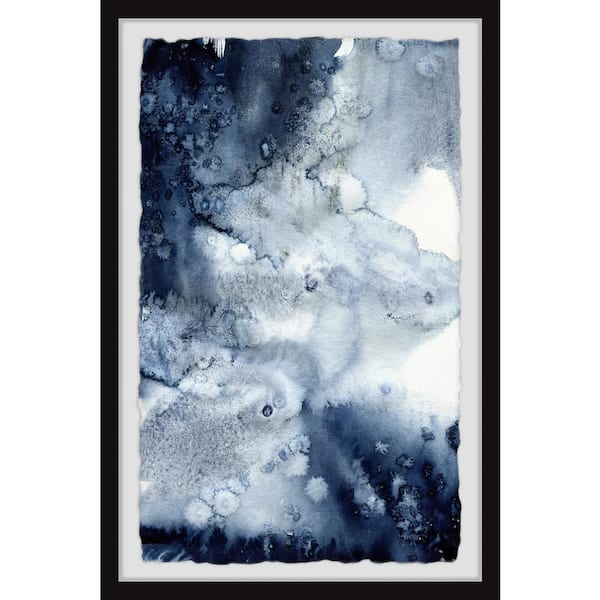This abstract art piece, displayed in a tall rectangular black frame, is characterized by a spectrum of dark to light blues, grays, and whites, creating a watercolor effect with a fuzzy, blended appearance. Dominating the piece are various hues of blue that appear dark and intense in the upper left corner and lower right corner, contrasted by lighter blues and whites towards the center. The central image features a band of white stretching through it and moving upward to the right. The white and blue splotches evoke thoughts of puffy clouds, snowflakes, or even a frost pattern, creating a dreamy and somewhat chaotic visual impression. This pattern, reminiscent of paint blobs or a spillage, includes circles bordered in blue with white interiors and blends intricately with darker shades. The frame includes a white matting, enhancing the depth and complexity of the artwork, inviting viewers to use their imagination to discern shapes within this modern, abstract composition.